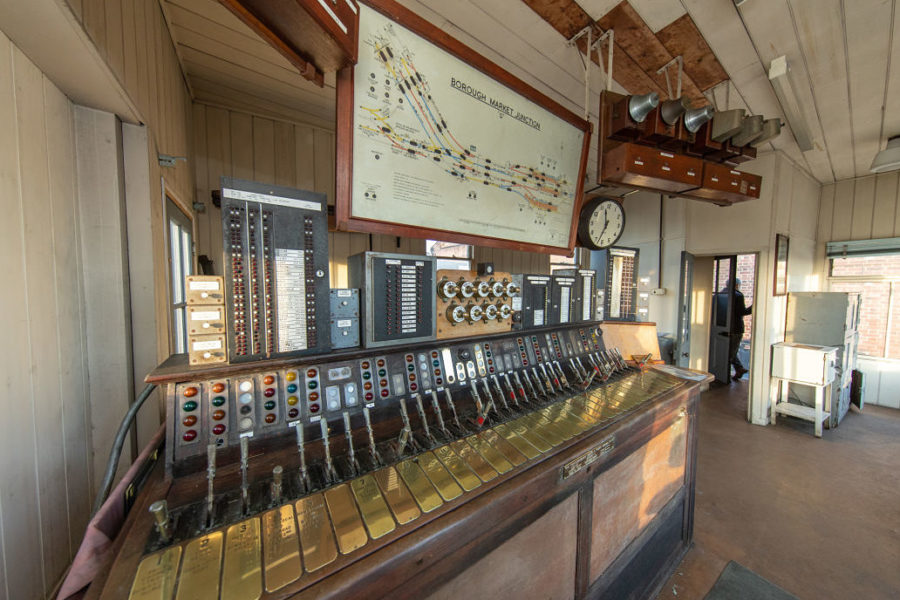The image showcases an interior of an old-fashioned train museum, dominated by a large, vintage control panel. The room features whitewashed wooden walls that give it a simple, yet historical feel. Central to the scene is the control panel, adorned with various colorful lights, buttons, and levers, along with numerous brass plates detailing its functions. Above the panel, a sign reads "Borough Market Junction," with a map displaying multiple railway tracks, suggesting this control panel is used to operate railway switches. Accompanying the panel are additional gadgets, boxes, and vents, indicative of its complex nature. There is a distinct, round clock on the wall and speakers hanging from the ceiling, perhaps used for announcements. A glass door provides a view of a brick building outside. The room's floor is made of dark brown concrete. In the background, a man is seen walking through a corridor, adding a touch of life to this vintage, yet possibly still functioning, operational setting.